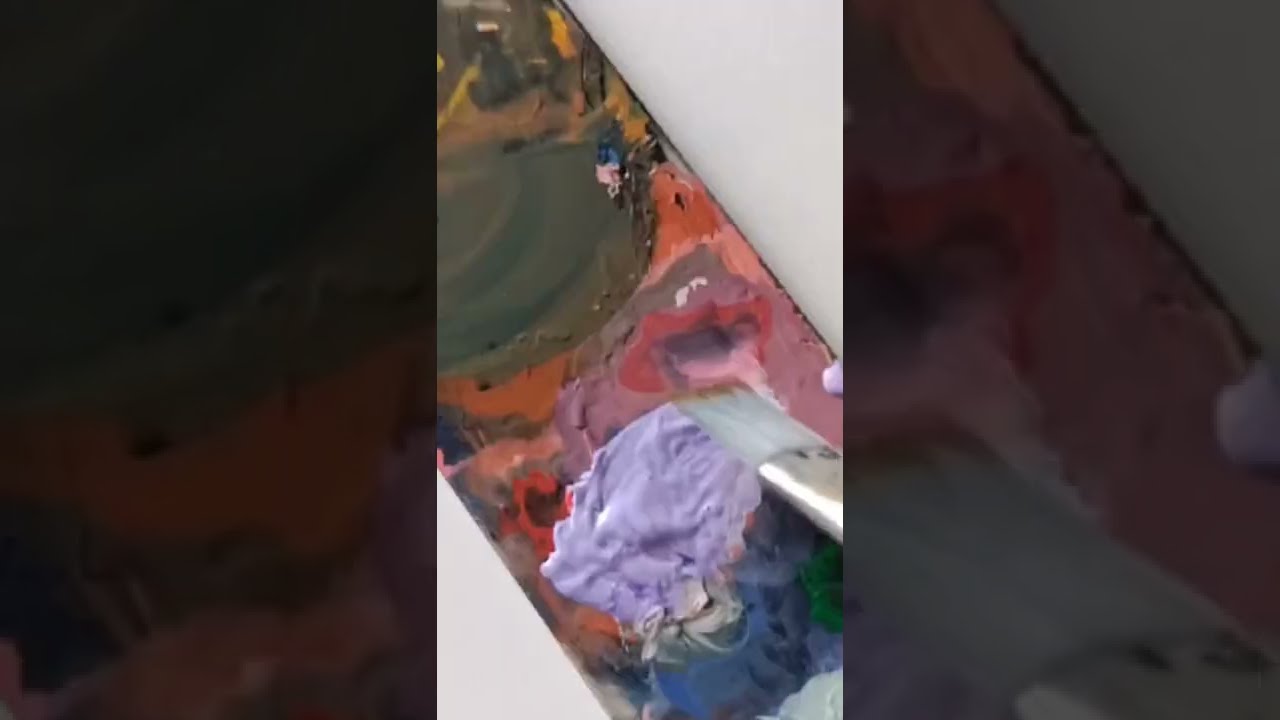The image captures a close-up view from above of a painter's palette positioned diagonally on a white table. The palette itself is a rectangular strip, likely made of cardboard or wood, covered in a multitude of paint splatters and spots, showcasing a spectrum of vibrant colors including brown, yellow, orange, red, purple, blue, and green. In the lower right corner of the image, a white-bristled paintbrush with a darker-colored tip is seen dipping into a light purple, lavender, or lilac paint. Surrounding this active dip are various blobs of other colors—deep blue below the purple, and mixtures of pinks and oranges and reds above it, with old dried brown paint at the top. The chaotic array of colors on the palette suggests that this is not the canvas itself but rather the surface the painter uses to mix and gather paint before applying it to their artwork.